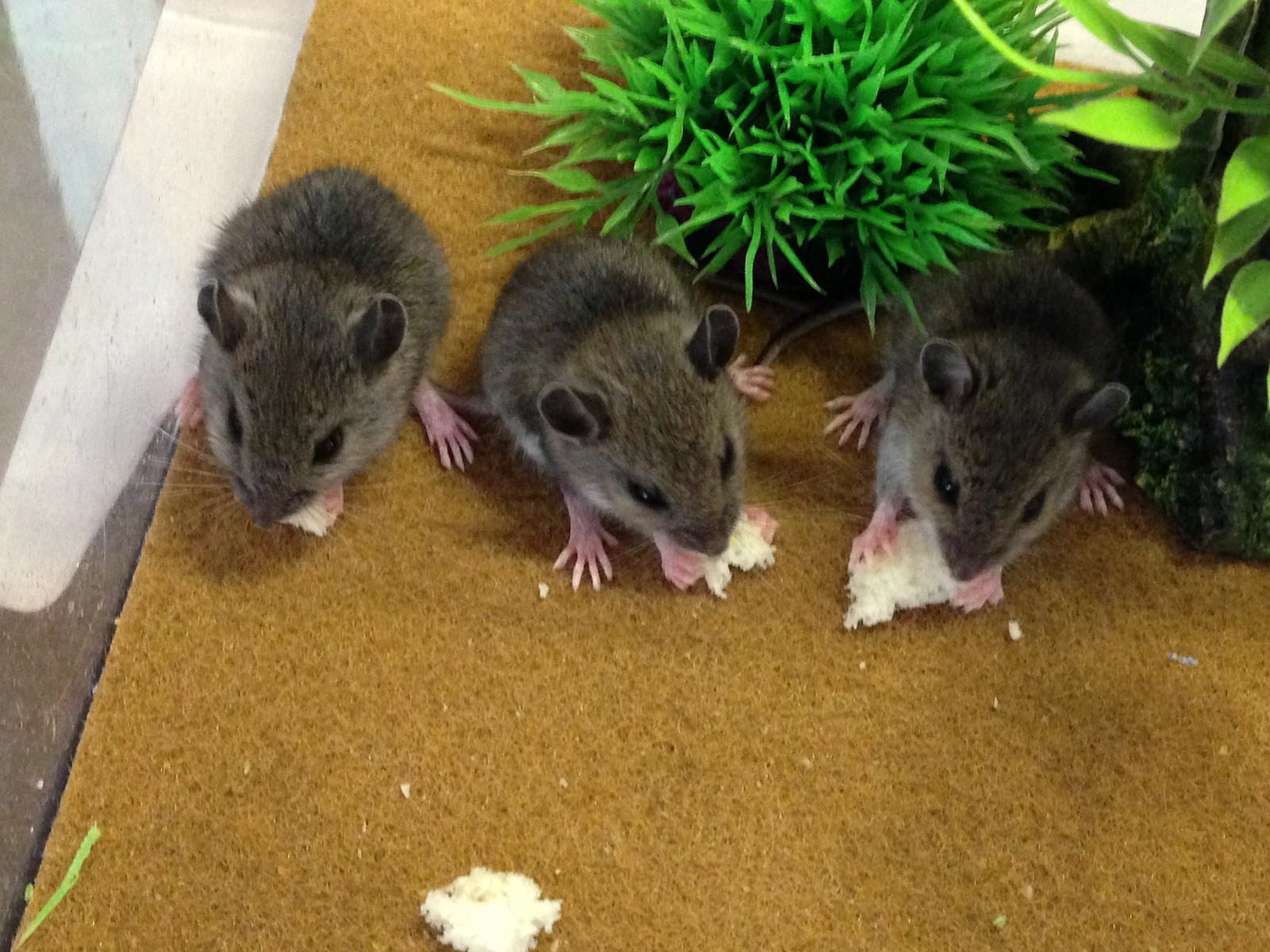The image features an overhead view looking down at three small, gray mice with dark gray fur that lightens towards their lower bodies. They are all nibbling on pieces of bread, with bread crumbs scattered around them. The mice are positioned on a brownish, slightly rough-textured rug or mat that appears to have small holes in it. Their paws and feet are pink. Behind the mice, there are bright green plants with varying shapes of leaves—some are pointy while others are more teardrop-shaped. The setting includes a white, painted wooden object in proximity, which might be part of a wall or ledge, and some gray concrete is visible to the side of the mat. All three mice seem calm and unafraid, suggesting they might be accustomed to human presence.